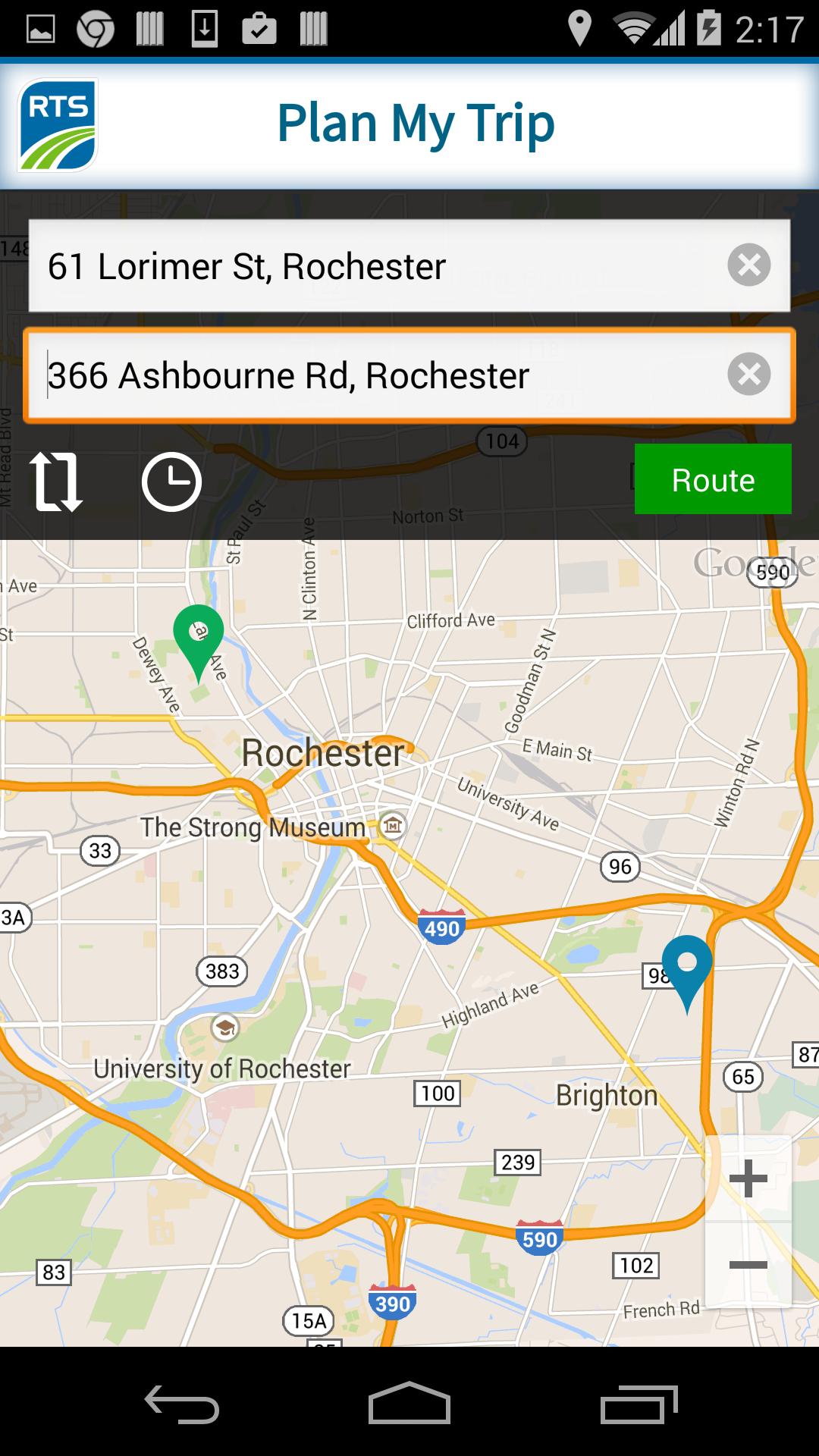This photograph, taken from a cell phone screen, features a detailed "Plan My Trip" display from an app. The lower part of the screen shows a map highlighting areas in Rochester, including landmarks such as the University of Rochester, the Strong Museum, and the neighborhood of Brighton. The map is rendered with roads in a yellowish-orange color. Two significant locations are marked with pins: a blue pin and a green pin. 

At the top of the display, there's an icon labeled "RTS," featuring a green road graphic on a blue background. Below this header, two addresses are prominently displayed: 61 Lorimer Street, Rochester, and 366 Ashbourne Road, Rochester. Further down the screen, the interface includes a symbol of two white arrows forming a rectangle, indicating directions, accompanied by a white clock icon. At the bottom, a distinct green button labeled "Route" in white text invites user interaction to finalize the trip route.